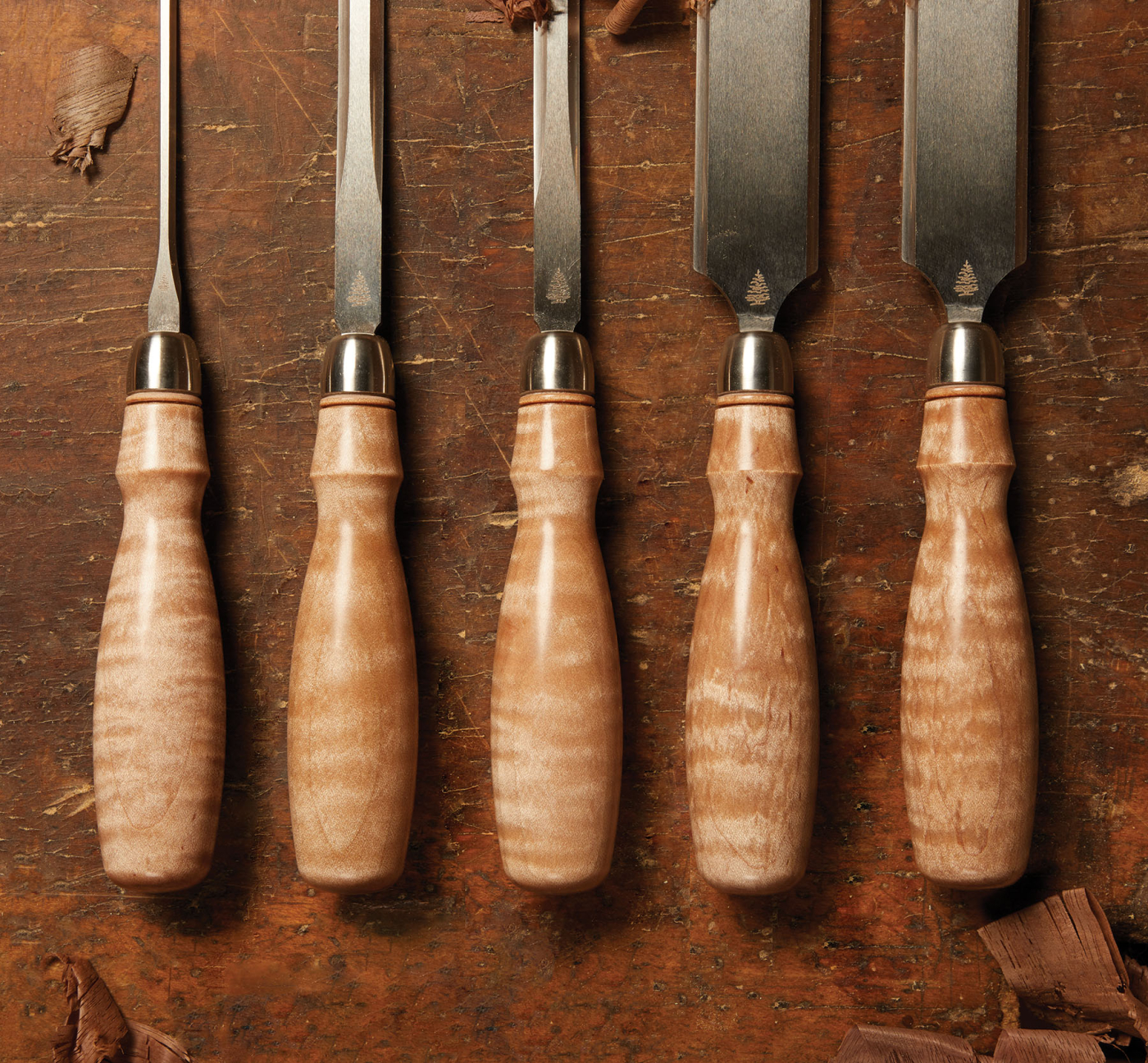This photograph features an array of five meticulously arranged woodworking chisels, each with a glossy wooden handle accented by a chrome keeper at the top. The chisels are systematically laid out on a wooden table, surrounded by small wood shavings, particularly noticeable at the top left and bottom right corners of the image. Starting from the left, the chisels vary in width, with the narrowest on the left and progressively increasing in size to the right. The chisels' reflective surfaces highlight their sharpness and pristine condition. The detailed grain of the wooden table and the chisels' handles, combined with their orderly placement, create an appealing composition that accentuates both their functionality and craftsmanship.